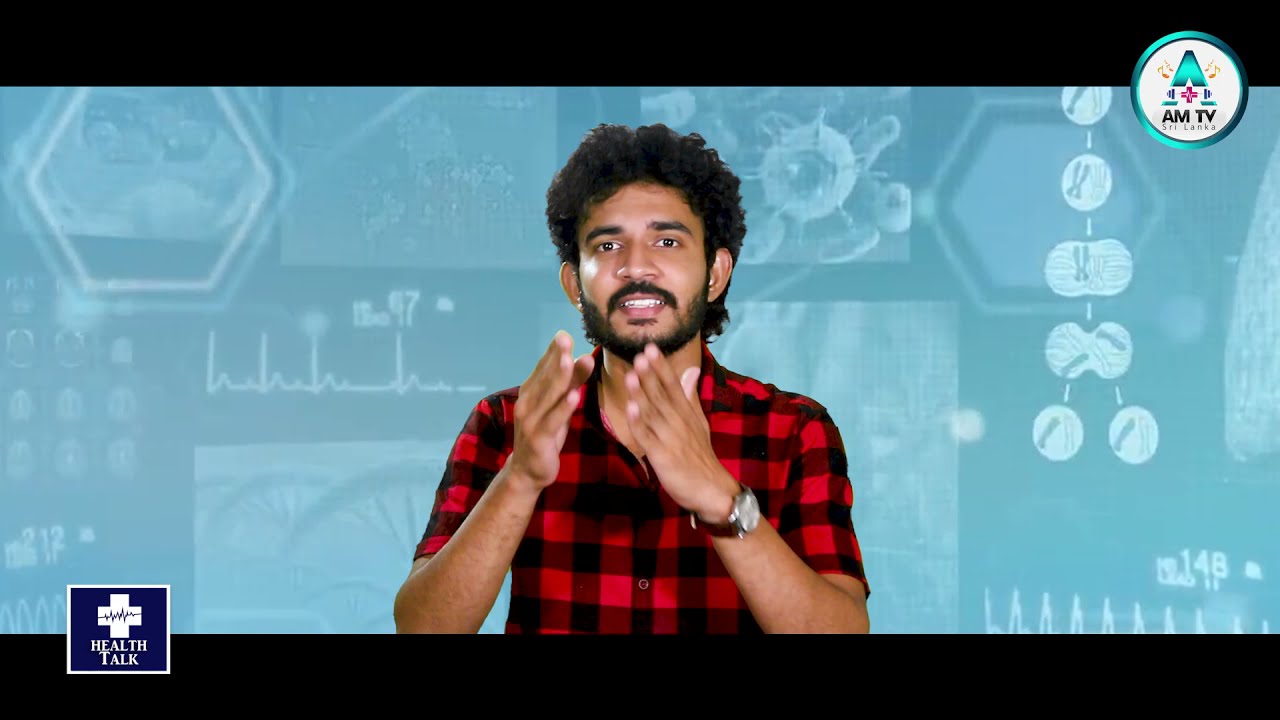The image is a screenshot from a TV show, possibly a live stream or a vlog, distinguished by the black borders at the top and bottom. In the center, a medium-skinned man, likely of Middle Eastern origin, is prominently featured. He has puffy curly hair, a well-groomed beard, and a mustache. He wears a short-sleeve, red and black plaid shirt and a watch on his left wrist, and is gesturing with his hands near his chin, appearing to speak directly to the camera, with his teeth visible.

The background is a mix of light and dark blue hues with white accents, showing generic medical imagery such as blood pressure numbers and molecular structures, enhancing the health-related theme. In the upper right corner, there's a white circular logo with a green border, containing medical symbols and the text "AMTV Sri Lanka." In the lower left corner, a blue circular icon with a white cross and a heartbeat line, labeled "Health Talk," further indicates the subject matter is focused on health discussions. The overall setup and design suggest this is a webcast or online health talk show.